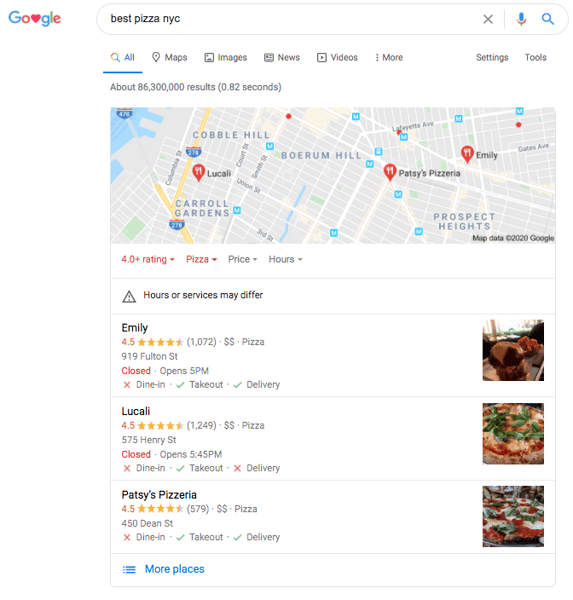In this image, we see a screenshot of a Google search result page set against a white background. In the upper left corner, the Google icon is prominently displayed, with a unique twist: the second "O" is replaced by a red heart. To the right of the icon is a search bar with the text "Best Pizza NYC" inside. Below the search bar, the navigation menu reads, from left to right: "All," "Maps," "Images," "News," "Videos," "More," "Settings," and "Tools."

A street map is displayed below, adorned with several red pins indicating the locations of various pizzerias in New York City. Notable locations include Lucali on the left, Patsy's Pizzeria to the right, and Emily further to the right. 

Beneath the map, search results are listed, complete with detailed reviews, ratings, and images. The first result showcases Emily with a rating of 4.5 yellow stars from 1,072 reviews. The listing includes two dollar signs to indicate price range, the category "pizza," and the address "919 Fulton Street." In red text, it is noted that the establishment is currently closed.